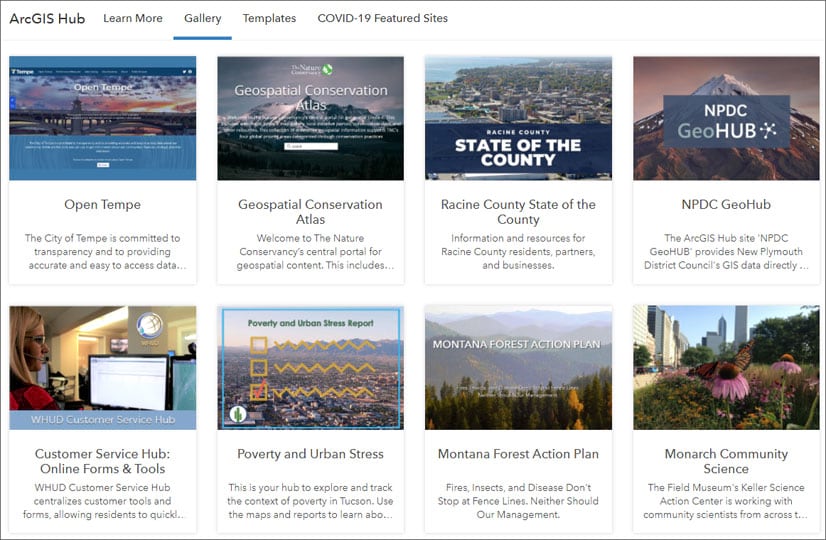On a white background, the webpage features the prominently displayed title "ArcGIS" in all capital letters. Below this, navigation links include "Hub," "Learn More," "Galleries" (all underlined in blue text), "Templates," and "COVID-19 Featured Sites."

The page is adorned with various sections and images. One section titled "Open Temp," accompanied by a picture, highlights the City of Tempe's commitment to transparency, stating, "As a City of Tempe, we are committed to transparency and to providing accurate and easy to access data…"

Another section features the "Geospatial Conservation Atlas," with a picture, welcoming users to "The Nature Conservancy Central Portal for Geospatial Content." The caption continues, “…This includes…”

Following this, the "Rakhine County State of the County" section provides information and resources for Rakhine County residents, partners, and businesses, again accompanied by an image.

The "NPDC GeoHub" section, featuring another picture, offers an array of information.

Highlighted next is the "Customer Service Hub," which includes online forms and tools, enriched by another illustrative image.

The section labeled "Poverty and Urban Stress" is repeated twice, both times including images and some relevant information on the topic.

Further down, sections on the "Montana Forest Action Plan" and the "Monarch Community Science" also offer thoughtful content paired with respective images.